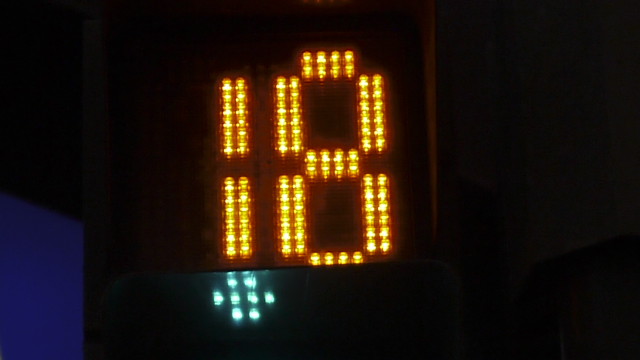The image features an illuminated sign displaying the number "18" against a dark background. On the left side, the number "1" is depicted as two vertical orange lines with a break in the middle, creating a segmented appearance. To the right, the number "8" is styled uniquely, composed of intersecting vertical and horizontal lines rather than the traditional circular form. Beneath the numbers, seven blue lights are arranged in a specific pattern, casting a subtle glow. In the bottom left corner of the image, there is a faintly visible blue rectangular shape, adding an extra layer of detail to the scene.